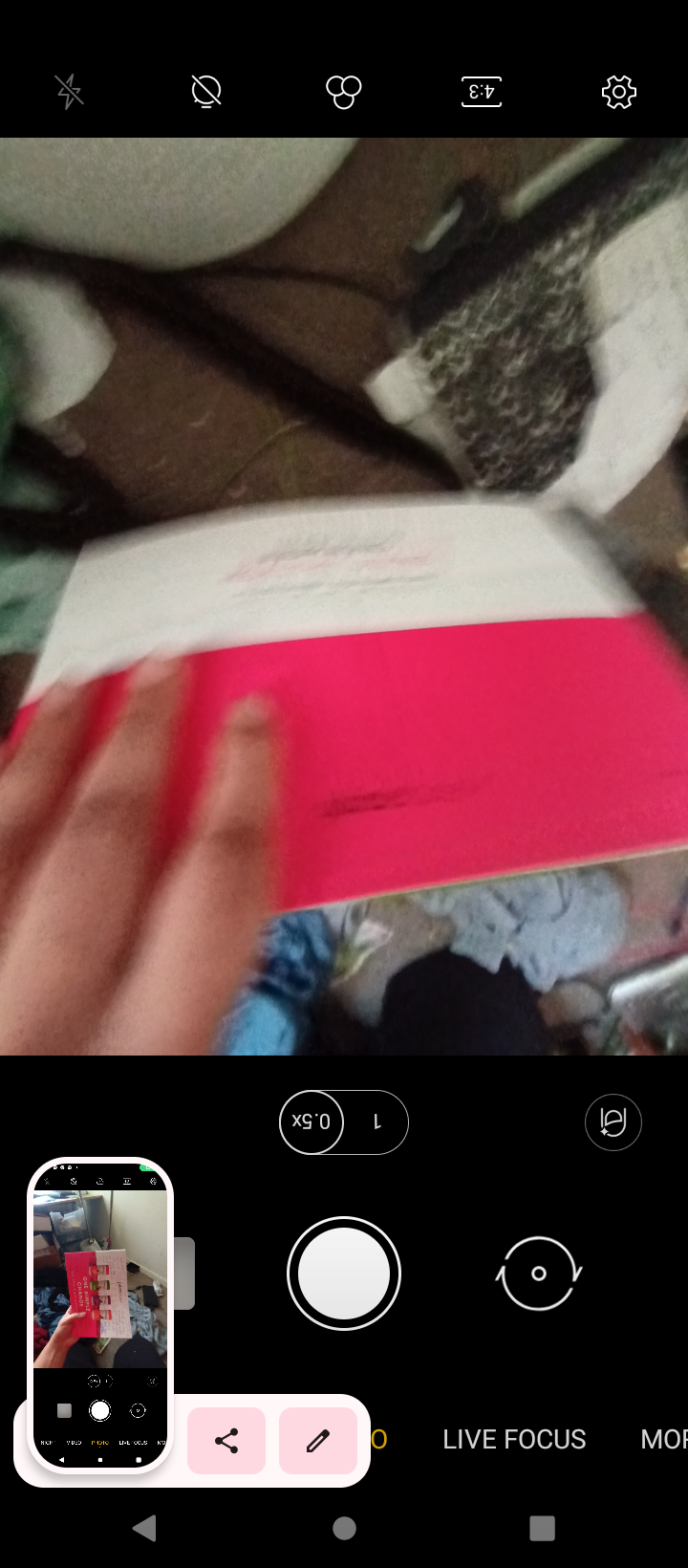A screenshot from a phone's camera app displays an image of a hand holding a red and white envelope, set against a cluttered background. The floor is visibly dirty, with various items scattered about, including a balled-up t-shirt or piece of clothing near the bottom. Above that, other miscellaneous objects are strewn across the floor. Interestingly, the camera controls on the phone screen are upside down, including the zoom indicator at the bottom. Adding to the oddity, there's a box in the bottom left corner of the screen showing another phone's screen, which also features the red and white envelope and shares a similar upside-down layout of controls.